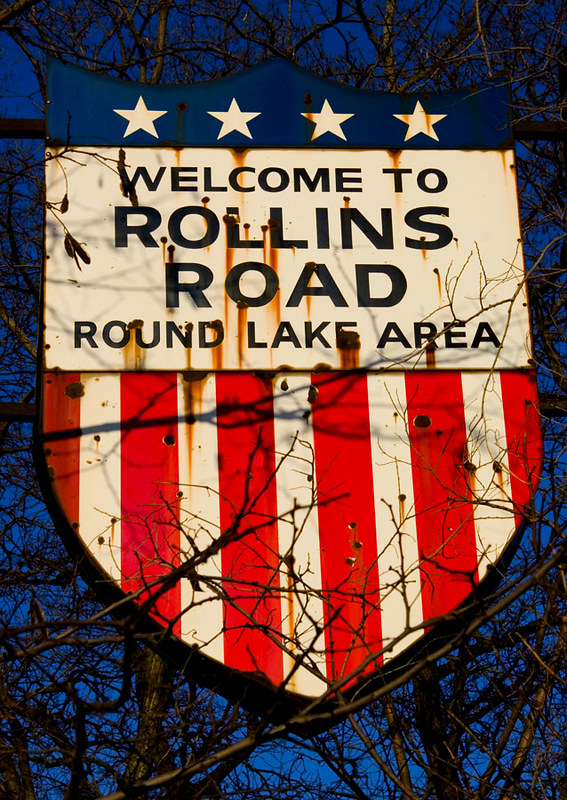The image depicts a rusted roadway sign resembling an American flag crest mounted amidst leafless tree branches against a deep blue night sky. The upper part of the sign features four white stars on a blue background, while below it, bold black letters on a rust-stained white rectangle read "WELCOME TO ROLLINS ROAD, ROUND LAKE AREA." The lower section of the sign showcases vertical red and white stripes, also marred by rust. This sign appears to be held up either physically or digitally among the tree branches, blending into the surrounding natural elements with some branches partially obscuring the sign.